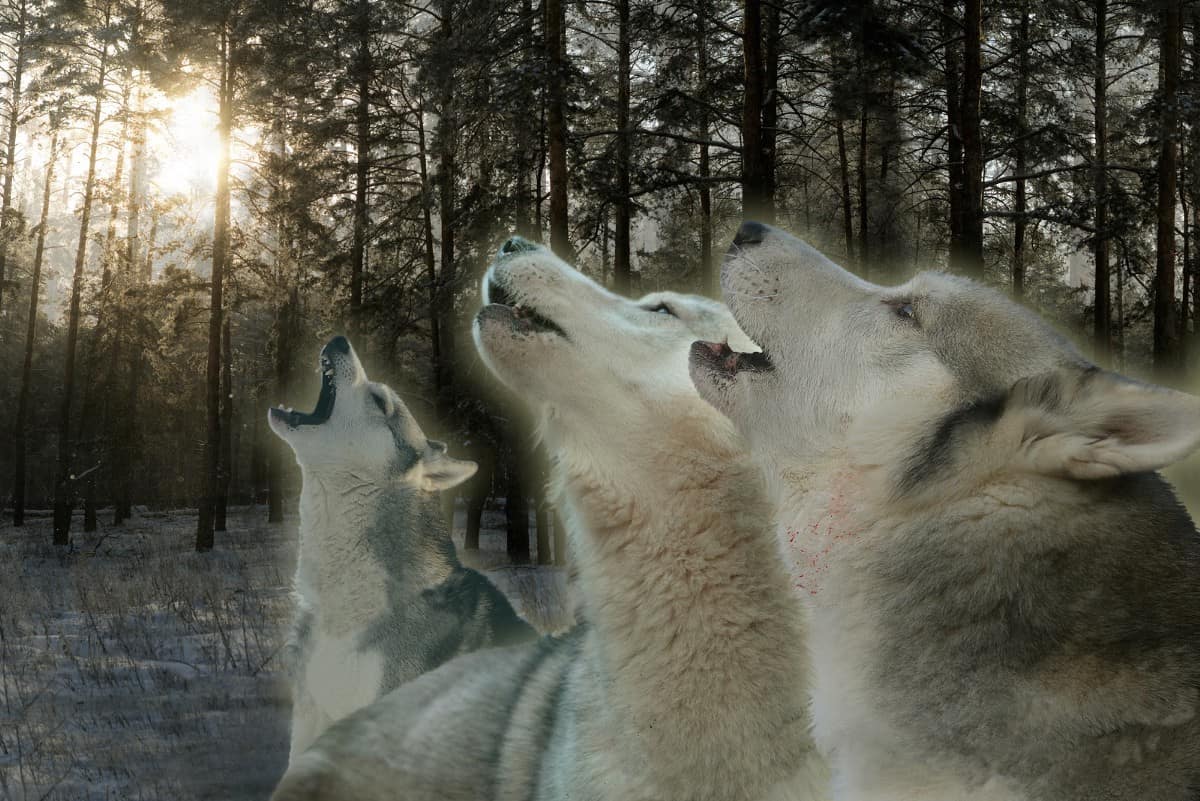In this evocative landscape image, the setting sun casts a dusky glow over a wintry forest with tall, leafless trees standing stark against the sky. The ground is covered in a sparse layer of off-gray snow, through which patches of grass occasionally protrude. Towards the left side of the image, the slightly obscured sun hints that dusk is approaching, its light glinting off the snow.

Dominating the scene from the middle to the far right are three wolves of varying sizes. They all have a mix of gray and white fur. The middle wolf, the smallest, has a noticeable abundance of white markings on its face and is caught mid-bark, its mouth wide open in an aggressive stance. The next larger wolf, positioned further right, also grey and white, is earnestly howling upwards. The largest wolf, closest to the viewer, shares this upward howl directed towards the left side, joining the chorus under the dimming sunlight. Together, these majestic creatures create a powerful tableau of nature's raw, unrestrained beauty.